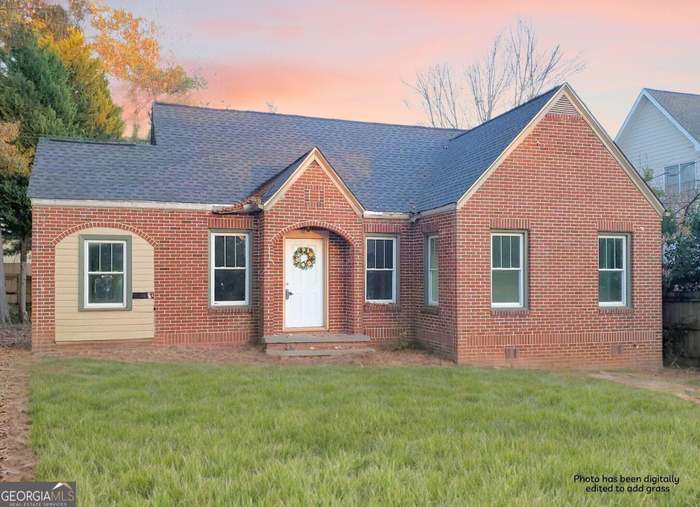This image depicts a large brick house with a white door adorned by a wreath and numerous windows, which are curtainless, allowing a clear view into the interior. The house features a gray roof with two prominent triangular peaks, one above the door and another on the front right side. The scene is set during what appears to be close to sunset, as the sky is tinged with pinks and blues, enhancing the tranquil ambiance. Notably, the grass shown in the photo has been digitally edited, as indicated by the annotation in the bottom corner from Georgia MLS, even though it looks lush and well-maintained. This digitally added grass surrounds the house, contrasting with a brown trail encircling it, and bordering what seems to be an unpaved walkway or driveway composed of dirt. In the background, a tree devoid of leaves towers behind the house, while another tree to the left showcases green and yellow foliage. On the right side of the image, the edge of a neighboring off-white house is visible.